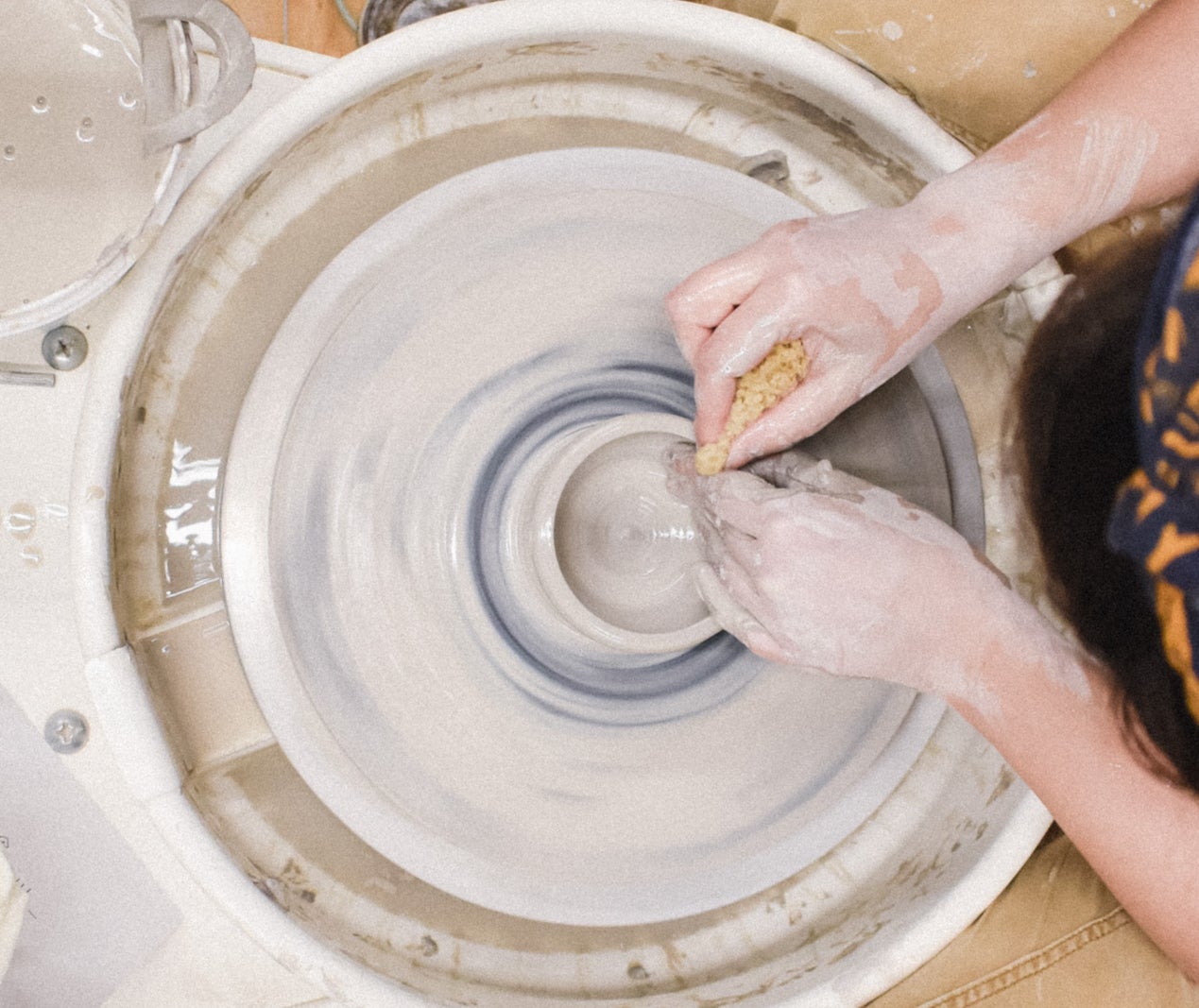In this detailed photograph, a person is meticulously crafting pottery on a spinning wheel. The central focus is the pottery wheel itself, which is a large white and gray circular device, adorned with two visible screws at the edge. The individual’s hands, smeared with wet, gray clay, expertly shape a pottery jar. Their right hand holds a yellow sponge, which they use to smooth the clay, while their left hand steadies the forming pot. The person is clad in a distinctively colored outfit, featuring a blue and orange shirt, with their dark-colored hair partially covered by a blue and gold material. They seem to be operating the wheel through a foot pedal, contributing to the wet and somewhat messy appearance of the workspace. The scene is captured from an overhead perspective, and the overall tone of the image is one of focused, artistic creation.